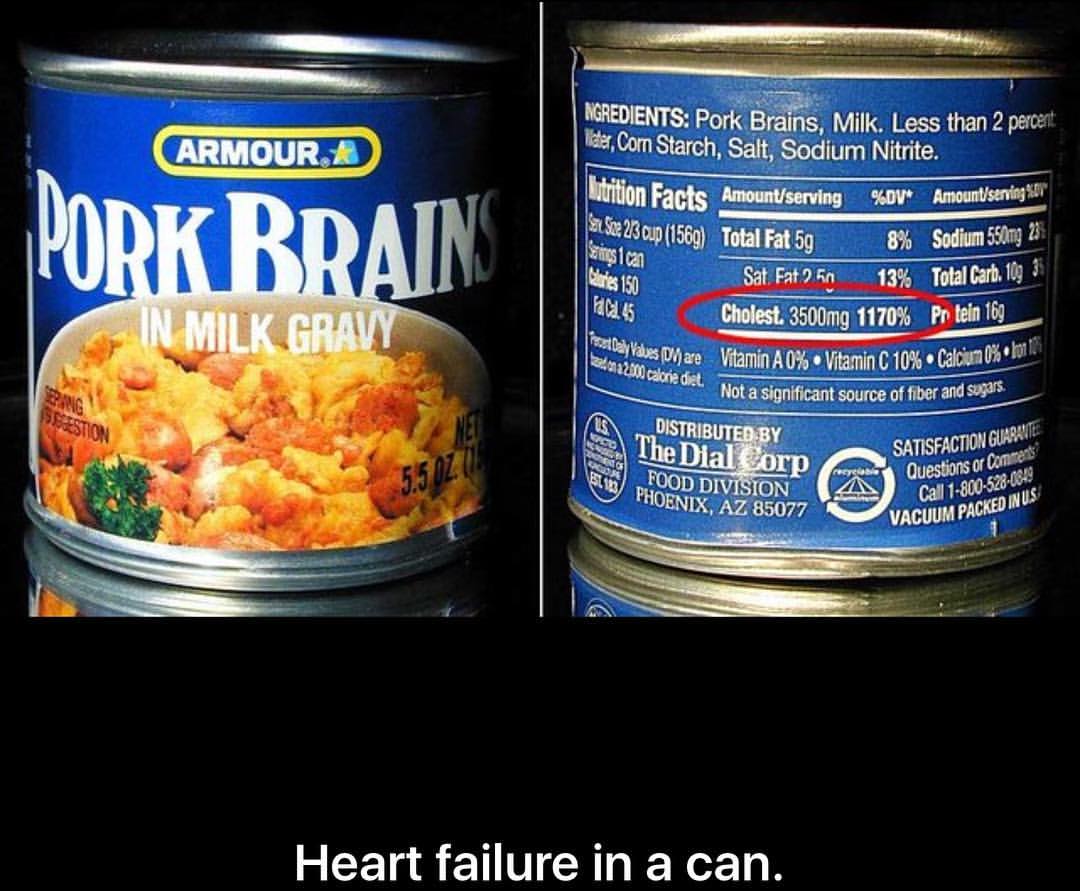This color photograph features a meme-like composition, with two images of a can side by side against a black background. The black areas are framed at the top and bottom of the photograph, enhancing the contrast. Written in white text at the bottom of the frame is the phrase "Heart failure in a can." 

On the left side of the image, the front of the can is prominently displayed. The can sports a blue background and showcases a bowl of food at the bottom, containing a mixture of yellow, orange, and green ingredients, all set in a white dish. The can is branded "Amour" with the product name "Pork Brains in Milk Gravy" clearly written in white text.

On the right side, the back of the can is presented. Here, detailed information is displayed, including a list of ingredients and nutritional facts, both written in white text. A starkly highlighted feature is a hand-drawn oval emphasizing the can's cholesterol content, which is a staggering 3500 milligrams, equating to 1178% of the recommended daily allowance. The can's bottom is noted to have a silvery tone in the left image, while appearing more golden in the right image, adding a curious visual disparity.

Overall, this detailed and striking image juxtaposes the literal packaging with the alarming nutritional content, underscoring the theme encapsulated in the meme caption.